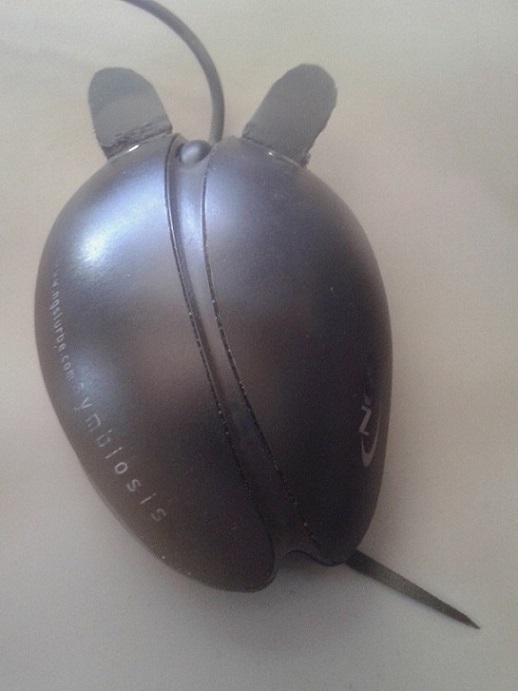The image features a close-up photograph of a wired computer mouse set against a gray background. The black, oval-shaped mouse has been designed to resemble an actual mouse, complete with two felt-like black ears attached to the front—one on each button. The left button is slightly more elongated than the right. Extending from the front of the mouse is its wire, resembling a tail coming out of a mouse's head. At the back, there is a small, spiky appendage suggesting an additional tail-like feature. The mouse appears to be well-used, with its white logo and text significantly worn off yet maintaining a reflective, polished surface. The photo is focused purely on the mouse, highlighting its animalistic design elements, such as the ears and tail, accentuating its playful appearance.